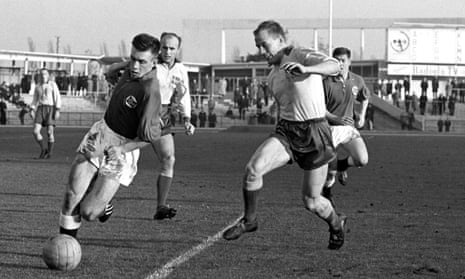This black-and-white photograph captures an intense moment in a soccer match, or "football" as known in Europe. In the foreground, two men are locked in competition near the ball. Both are donned in traditional soccer uniforms, featuring cleats and short shorts. One player, clad in a white t-shirt, is poised to kick the ball, while his opponent, wearing a black t-shirt, moves in to challenge and possibly steal the ball away. Behind them, additional players can be seen running towards the action, diligently maintaining their positions on the pitch. Spectators dot the background, their eyes fixated on the unfolding game. A visible white line runs down the center of the field, implying the midfield line. Additionally, a large building looms in the distance, adding to the historical and communal atmosphere of the scene.